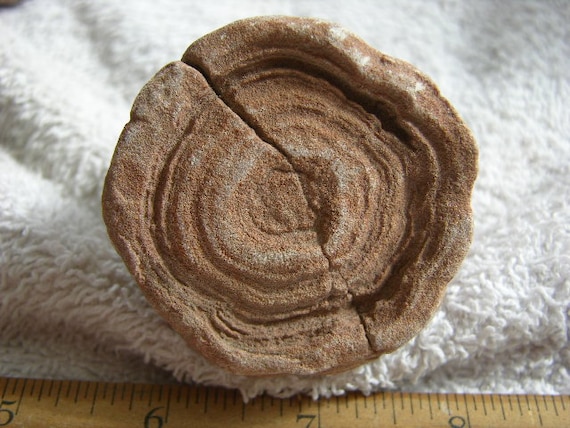The photograph depicts a circular object, about 2 inches in diameter, resting on a white, fuzzy towel or carpet. Positioned at the bottom of the image is a light tan ruler, partially visible and marked with the numbers 5 through 9 in black, suggesting the photo's width is 4 inches. The object itself appears to be a round, possibly cracked, rock or petrified wood, showcasing intricate layers or rings inside, hinting at its natural formation. Its coloring is predominantly brown with hints of bronze and silver, giving a textured, layered appearance that could suggest it’s a sedimentary stone or a handcrafted item. The scene is set indoors, with the ruler aiding in providing size reference for the object.